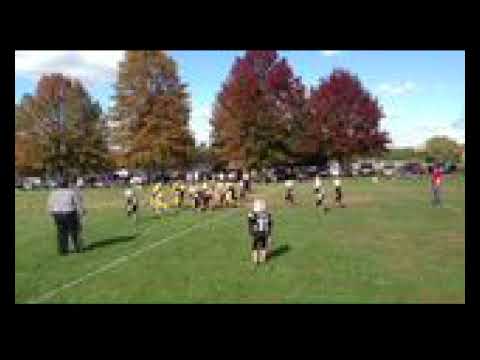In this extremely low-quality, pixelated image, we see a grassy sports field bordered by a black border on the top and bottom. The setting is outdoors, likely in the middle of the day, with a blue sky dotted with clouds and a background featuring four large trees in dark fall colors such as orange, maroon, and brown. 

The field is green, and in the center, a group of kids is playing, possibly engaged in a football or soccer game. The kids appear to be wearing white helmets and black jerseys. Toward the left side of the image, there's an adult, seemingly the referee or coach, dressed in a gray sweater and black pants. To the right, another person stands wearing a red shirt. Some bleachers can be seen with people sitting on them, but due to the poor quality, intricate details are hard to distinguish. Also, some buildings are faintly visible in the far background. There is no text visible anywhere in the image.